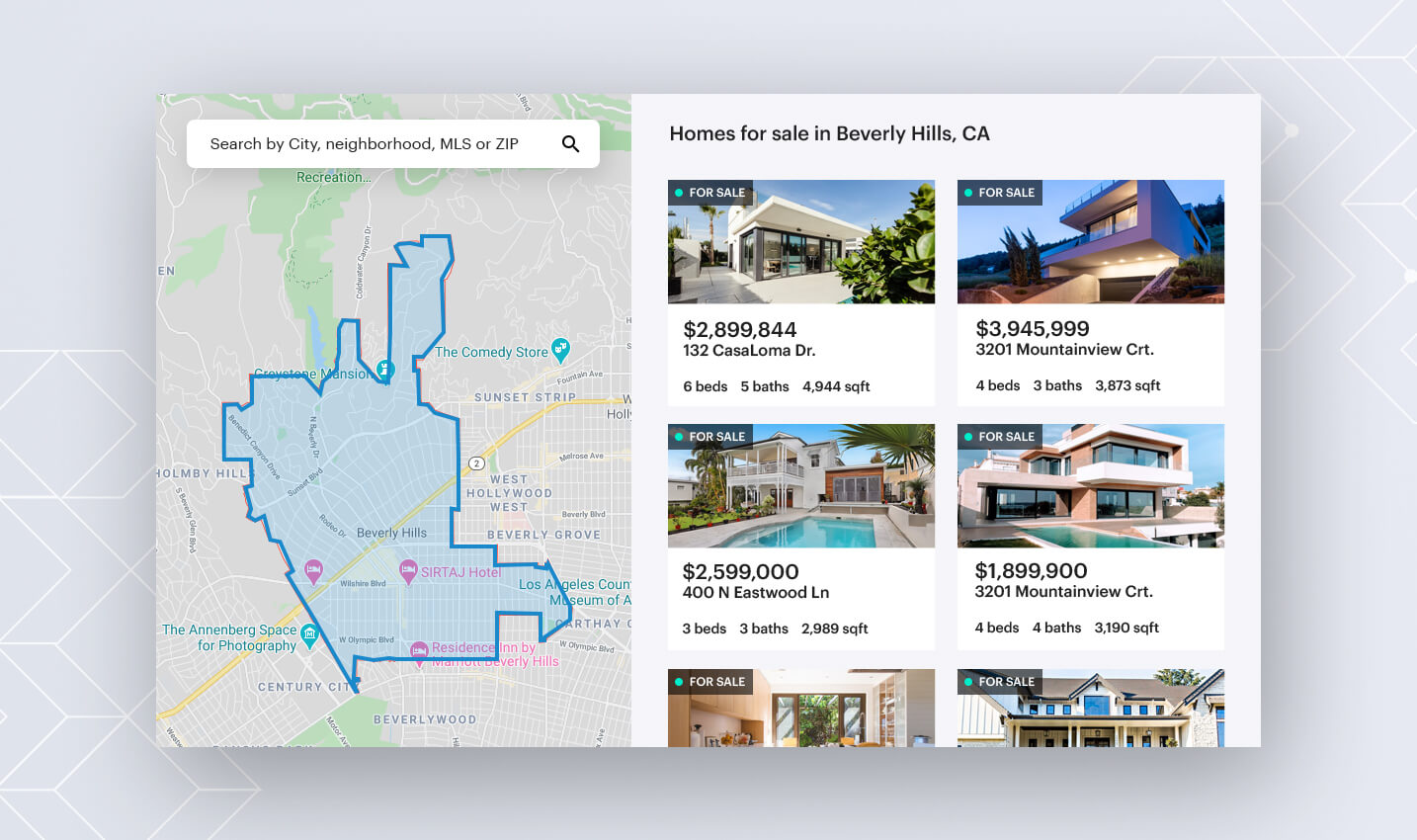Here's a detailed and cleaned-up caption for the described image:

---

The screenshot depicts a web page featuring a real estate map of Beverly Hills, California. The background is a sleek gray, adorned with subtle geometric patterns in white lines at the bottom left and top right corners. Dominating the center-left portion of the screen is a map with a highlighted blue area, showcasing the town of Beverly Hills. Within this blue-outlined region, three pink markers indicate various hotels, including the Sirtaj Hotel and the Residence Inn by Marriott Beverly Hills, with a third, unnamed marker. Just outside the blue area is the Annenberg Space for Photography and the Los Angeles County Museum (with only the letter "A" visible). Another marker points to The Comedy Store near the Sunset Strip, and "West Hollywood West" is labeled twice just outside the blue area.

On the right half of the screen, there are six images of homes for sale, each boasting modern architecture. The title at the top reads "Homes for Sale in Beverly Hills, California." The first property listed is priced at $2,899,844, located at 132 Casa Loma Drive. It features six bedrooms, five bathrooms, and spans 944 square feet. The remaining properties vary slightly in price and size but exhibit similar contemporary designs and layouts.

---